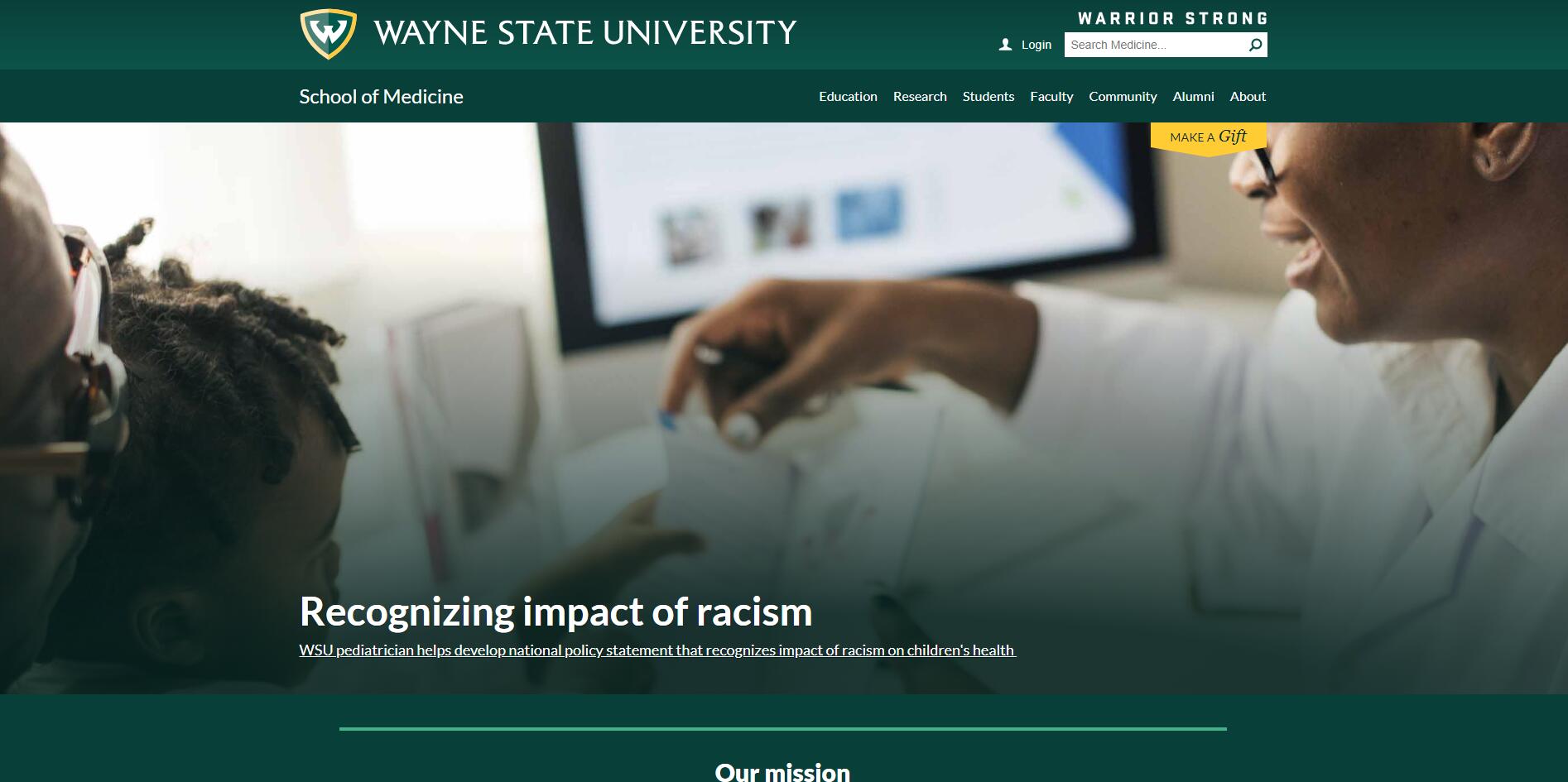Here is a descriptive and detailed caption based on the provided voice description:

---

This screenshot depicts the homepage of Wayne State University's School of Medicine website. The background features a soothing light green color. At the top of the page, a prominent banner displays the Wayne State University logo, consisting of a stylized 'W' enclosed within an orange-and-gold shield. Adjacent to this logo, there is a login section and a search box specifically for "Search Medicine." Above the search box, the phrase "Warrior Strong" is prominently highlighted.

Beneath the top banner, a secondary section identifies the "School of Medicine," accompanied by menu navigation items including "Research," "Students," "Faculty," "Community," "Alumni," and "About." Just below the "Alumni" and "About" links, there is a gold-colored banner that reads "Make a Gift," likely a clickable button for donations.

Dominating the central area of the page, a heartfelt photograph showcases a Black technician or doctor attentively engaging with a young girl patient. Below this touching image, a headline reads: "Recognizing the Impact of Racism. The WSU pediatrician helps develop a national policy statement that recognizes the impact of racism on children's health." The page concludes with a mission statement at the very bottom, underscoring the institution's commitment to their cause.

---